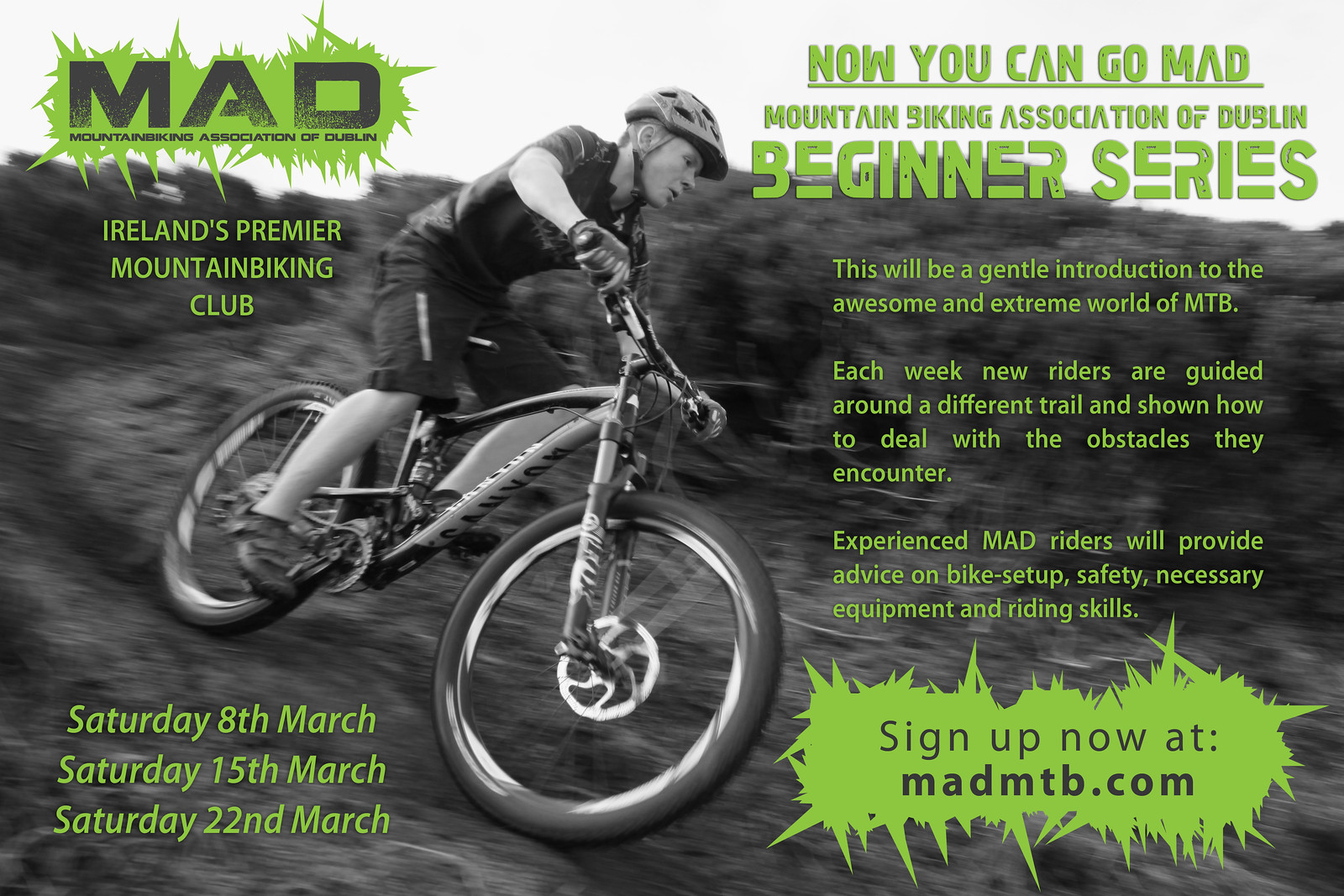The image prominently features a man riding a mountain bike down a trail, with a dark, gray-toned background that includes a dirt path and some hills. The rider is equipped with a helmet, emphasizing safety. The primary focus of the image is on promoting the Mountain Biking Association of Dublin (MADD), identified as Ireland's premier mountain biking club. The text written in bright green provides key details: the club's beginner series happening on Saturday 8th March, Saturday 15th March, and Saturday 22nd March, encouraging new riders to experience mountain biking in a guided, safe manner. Experienced MADD riders will be present to offer advice on bike setup, safety, necessary equipment, and riding skills. Additional text highlights "Now You Can Go MADD" as part of the promotional call to action. At the very bottom left corner, the website for more information and sign-up is listed as MADDMTB.com.